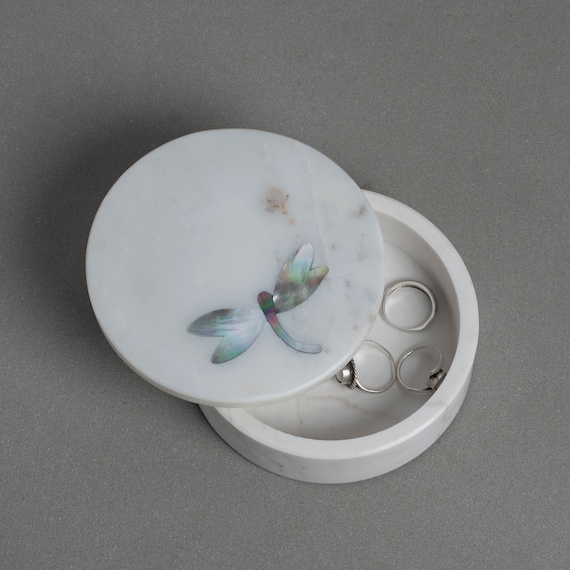The image depicts a small, round jewelry container with thick white walls, which appear to be made of marble or a hard plastic. The container sits on a medium-toned gray, textured surface. Inside this inch-and-a-half tall bowl are three small silver rings, reminiscent of elegant costume jewelry. The container’s lid, partially shifted to one side to reveal the rings, features a striking, ceramic dragonfly embellishment. The dragonfly boasts a colorful rainbow effect with a light blue body, pink-colored tips, and light teal wings. The overall scene exudes a visually appealing charm, with the marble-like material of the container and lid adding a touch of sophistication.